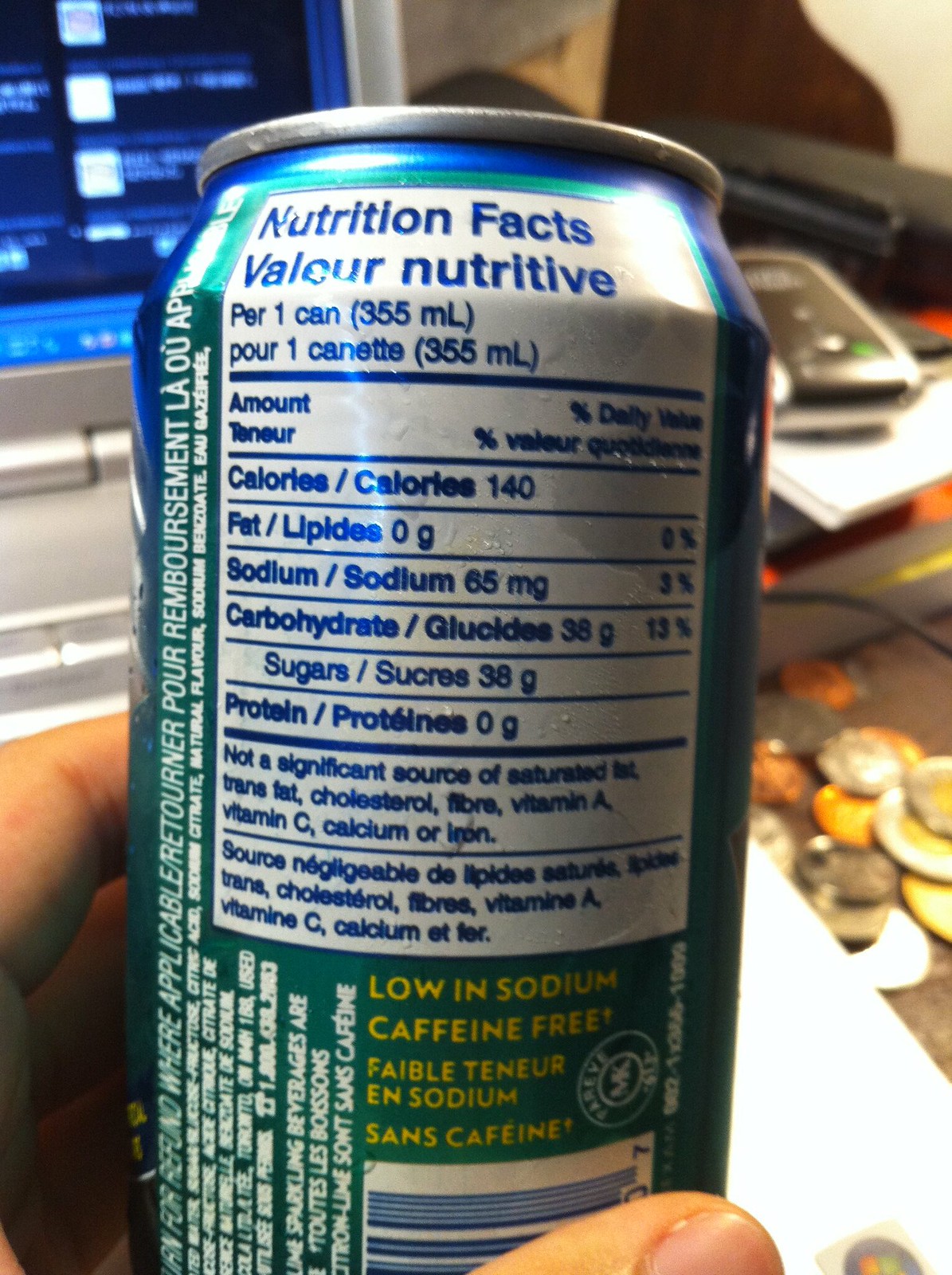The image features an up-close view of a person holding a turquoise aluminum can with condensation, focusing on the nutritional facts label on the back. The can is primarily green with blue accents, possibly indicating a Sprite or 7-Up drink. The nutritional information is presented in both English and French within a white rectangle that reads "Nutrition Facts" and "Valor Nutritif." Below it, in yellow text, it notes "Low in Sodium, Caffeine Free," and includes a sideways barcode with blue lines. The person is holding the can with their left hand against a backdrop that includes an open silver laptop on the left side of the frame, showing a portion of its screen. To the right of the laptop, there is a pile of coins, likely not American, suggesting a variety of denominations. The scene appears to be set on a desktop or countertop with other objects, possibly including a phone, adding context to the surroundings.